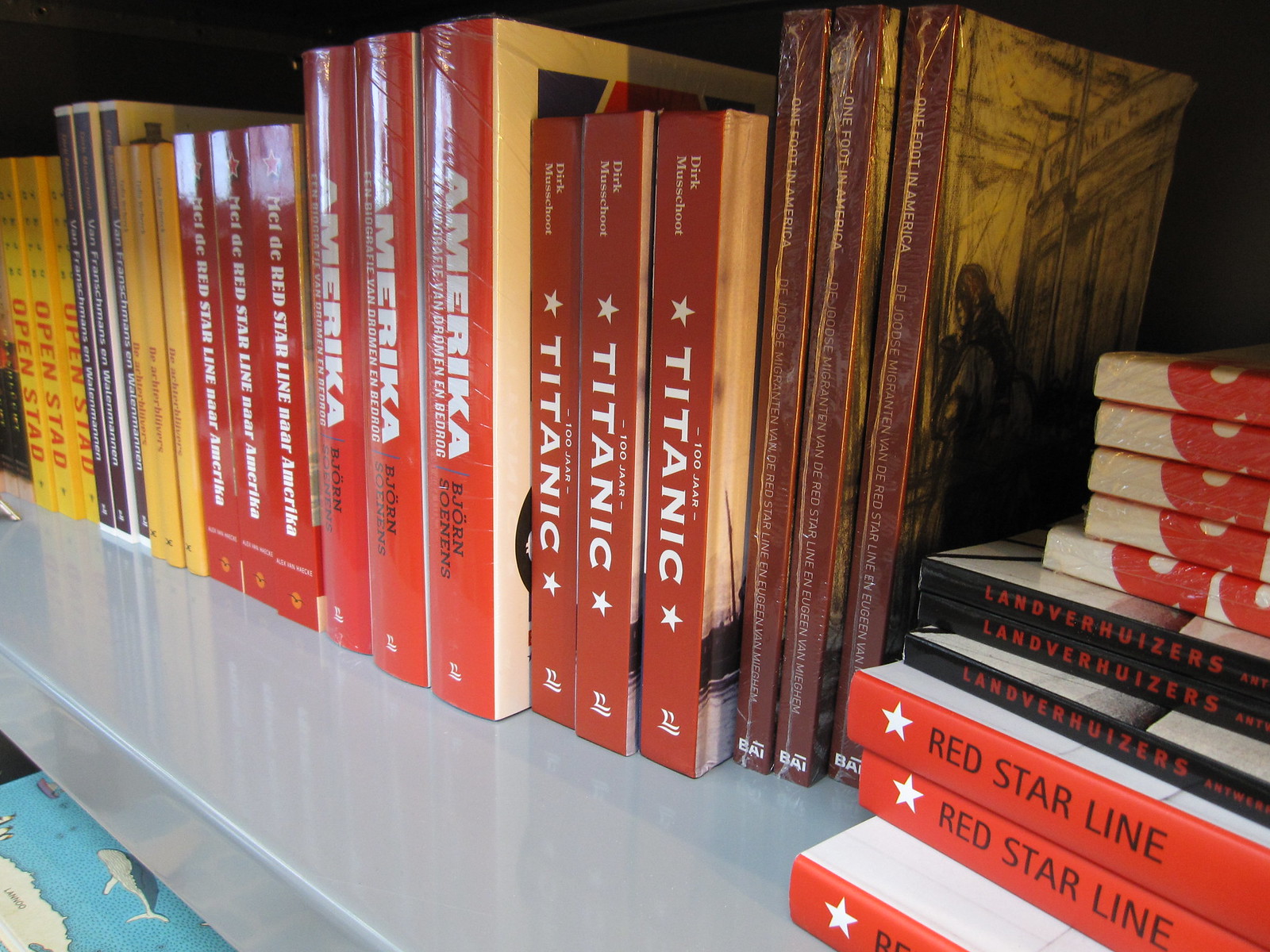This image is a detailed close-up of a light gray bookshelf, likely taken in a bookstore or library. The shelf prominently features a variety of books with spines predominantly in shades of red, orange, and yellow. The background is completely black, ensuring that the books are the sole focus of the image. On the bottom right corner, there is a pile of books. Among them, there are multiple copies of a book with red spines, a white star icon, and the title "Red Star Line" in black capital letters. Above this, there's a book titled "Landver Hoosers" with black and orange coloring. To the left, three copies of "Titanic" books are visible, alongside a book titled "America" with a distinctive 'K' at the end. A yellow-covered book titled "Open Stad" is also noticeable. Some of the books are taller and thinner with brown and yellow designs, potentially linked to Titanic themes as well.